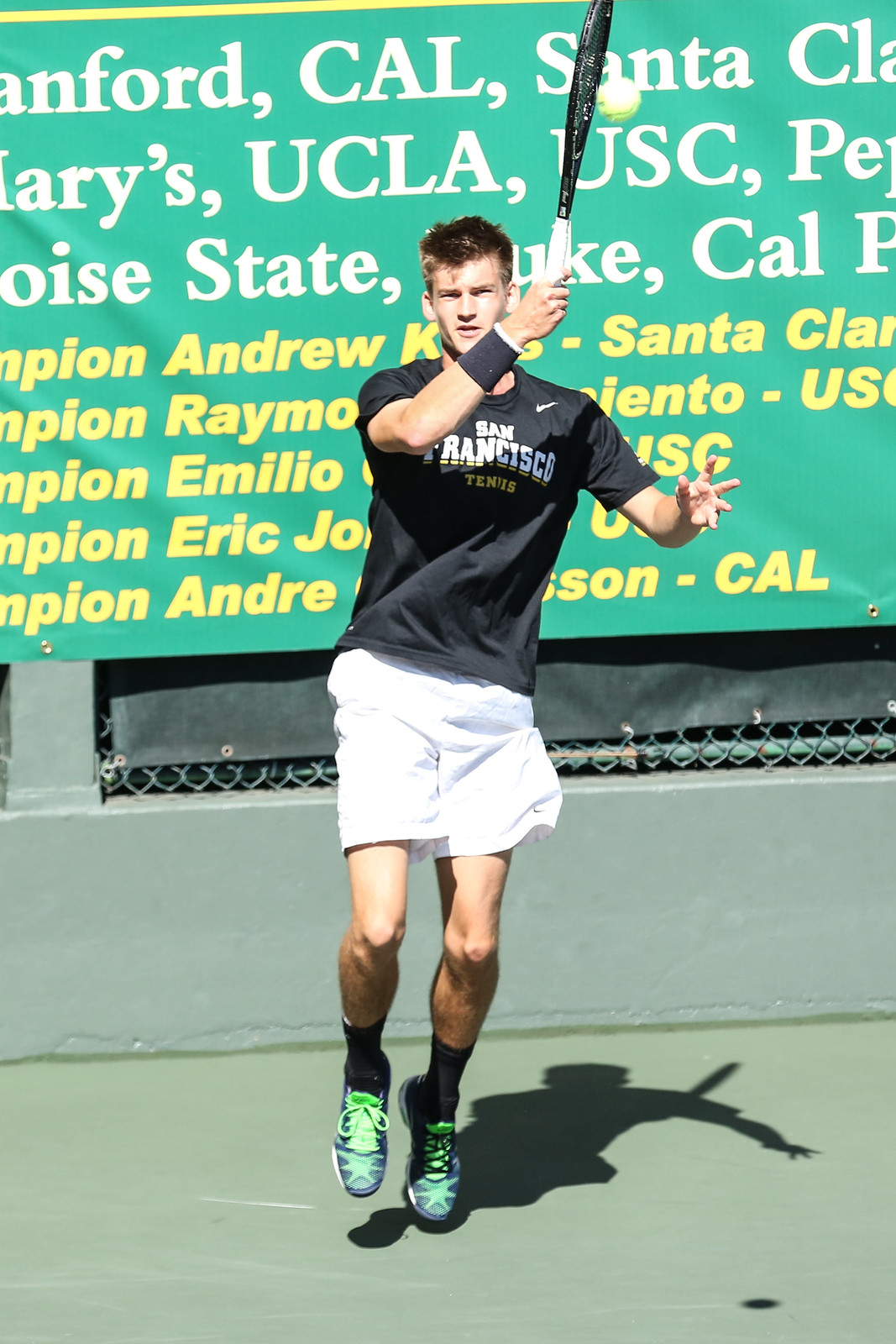The image depicts a college-aged student playing tennis on a green court. The student is tall with short black hair and is captured mid-swing, hitting a yellow tennis ball above his head with his right hand. He is dressed in a black T-shirt that reads "San Francisco Tennis" with a small Nike symbol on the left shoulder, paired with white shorts and black and green tennis shoes. The background features a green banner listing various colleges such as Stanford, UCLA, Boise State, along with a partially obscured list of champions, including names like Andrew from Santa Clara. The banner also displays a thin yellow stripe and uses white and yellow lettering.